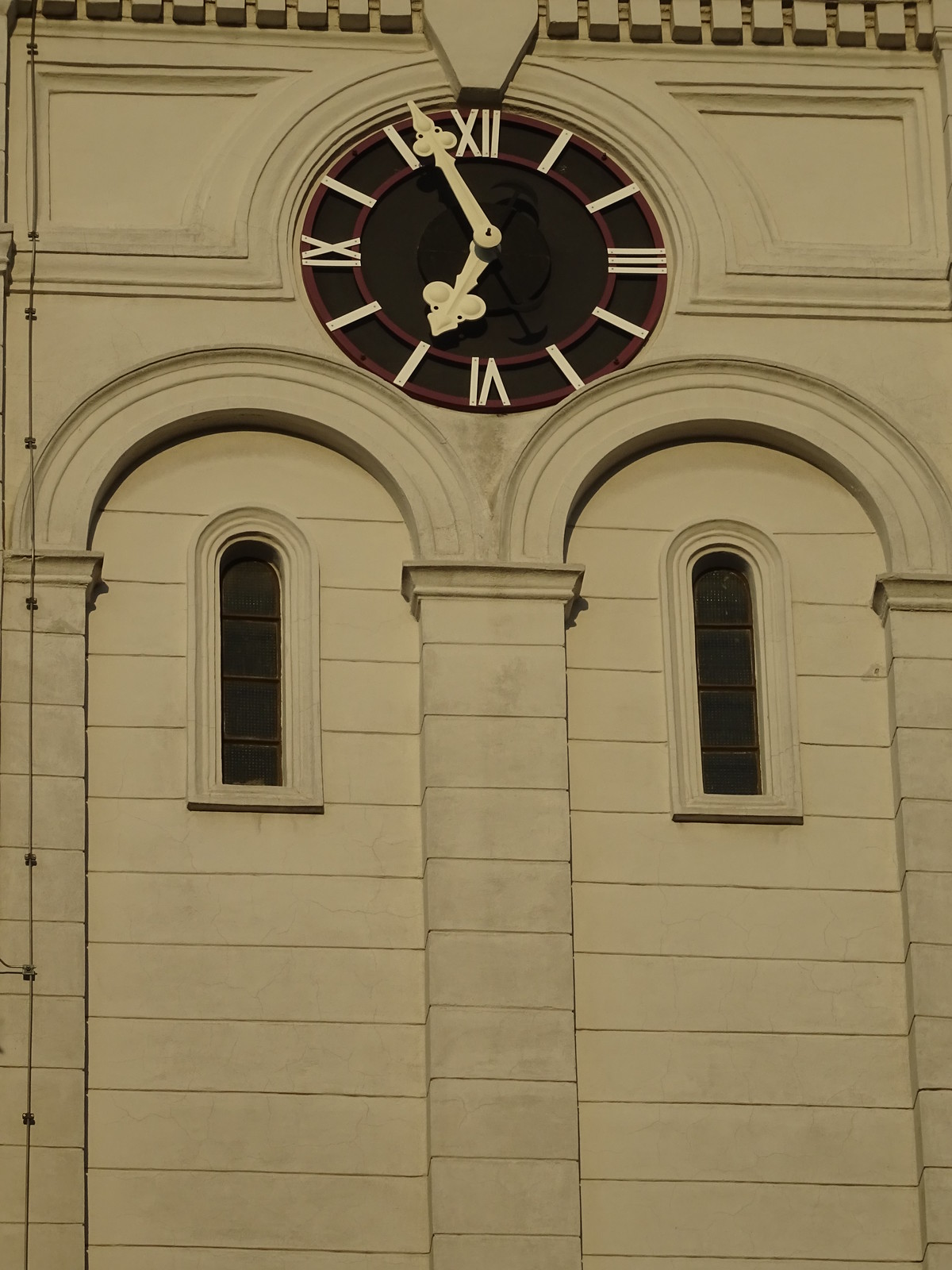This photograph captures a detailed view of a beige building seemingly made from cement or concrete blocks. The image focuses on a prominent clock, suggesting the building might be a part of a clock tower. The tower face features small, narrow, arch-shaped windows with clear glass, flanked by a symmetrical arrangement on both sides. Two arch-like structures resembling rainbows are visible, attached to posts, framing these windows. The clock, positioned at the top center, is circular with a black face and a dull red border. It displays white Roman numerals, and the time is approximately eight minutes to seven, indicated by slim, pointed hour and minute hands. A distinct rectangular architectural detail surrounds the clock, which includes curved and straight lines, adding depth to its setting. Additionally, a wire is seen climbing up the facade, though its purpose is unclear.